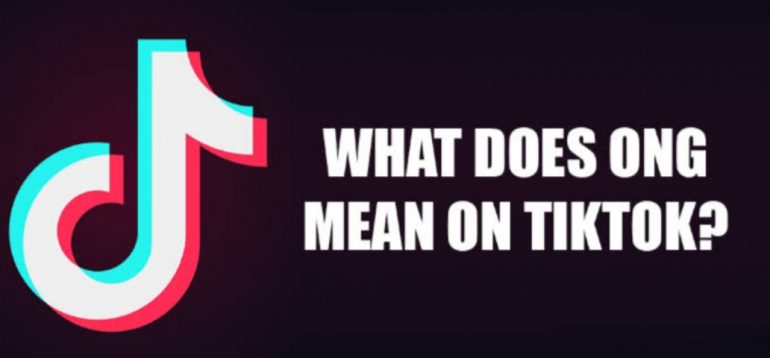The image features a black rectangular background, oriented horizontally. On the left side, there's a prominent TikTok logo, which is a combination of white, green, and red colors. To the right of the logo, in large, all-capital white letters, the text asks, "WHAT DOES ONG MEAN ON TIKTOK?" followed by a question mark. 

The text is positioned towards the middle-right of the image and stays well-centered, leaving a slightly larger amount of negative space at the top compared to the bottom. The fonts used are clear and easily readable even when the image is enlarged, maintaining a high resolution. Overall, the design is clean and balanced, with the TikTok logo nearly touching the left edge of the image but maintaining an elegant spacing, ensuring the viewer's focus is naturally distributed without any discomfort.

The color palette is minimal, comprising only black, white, green, and red, which contributes to the simplicity and clarity of the design. There are no additional elements or distractions within the image, making its message direct and aesthetically pleasing.